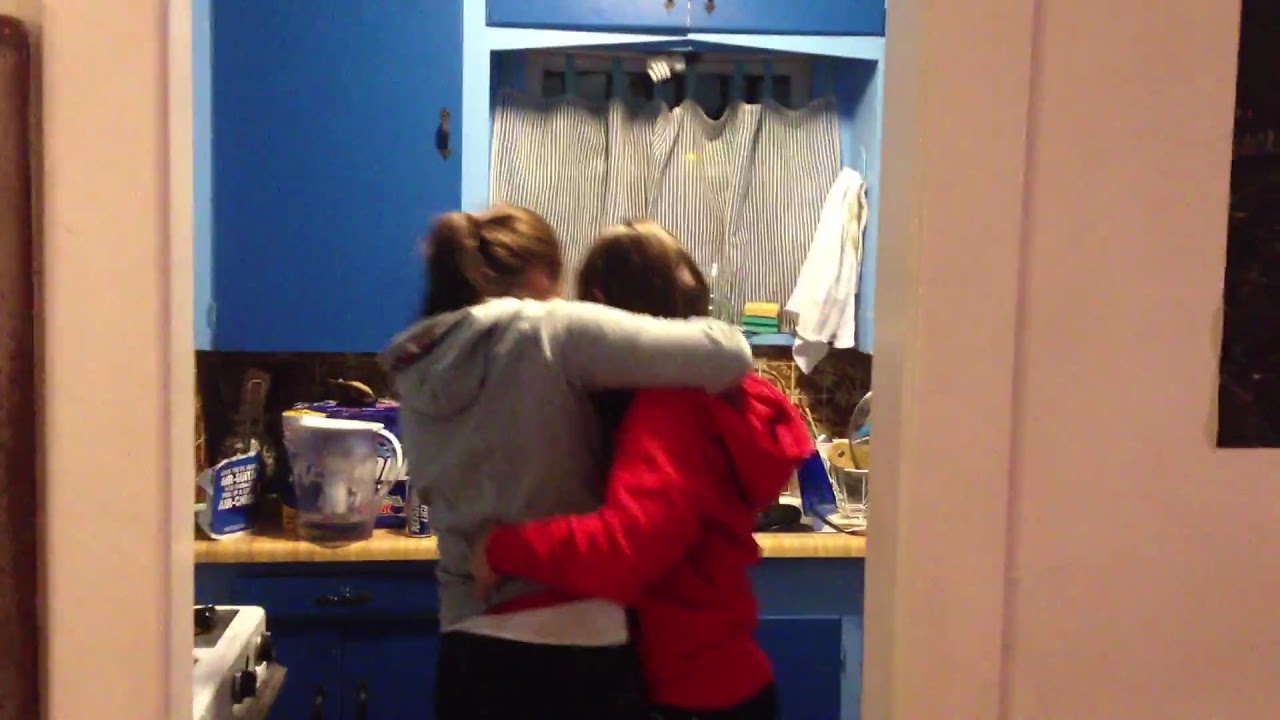The photograph captures the interior of a kitchen with two women at the center of the room, their backs to the camera, engaging in what seems like a heartfelt embrace. The woman on the left, identifiable by her brown ponytail and gray hoodie over a white t-shirt, has her hand placed gently on the shoulder of the woman on the right. The woman on the right, with her brown hair down and dressed in a red hoodie, has her hand around the waist of the first woman. Both are wearing black pants.

Behind them, the kitchen features a counter with a butcher block surface cluttered with various items, including a water pitcher, a towel, and a beer can. Cabinets above the counter are a mix of dark and light blue, some of which have their doors open. There are also white curtains with gray vertical stripes adorning the window above the countertop, through which a set of blinds is visible. In the bottom right corner of the image, part of a white stove with black knobs peeks into view. The overall setting is cozy but filled with numerous objects, enhancing the lived-in feel of the space. The pink walls add a warm, contrasting background to the scene.